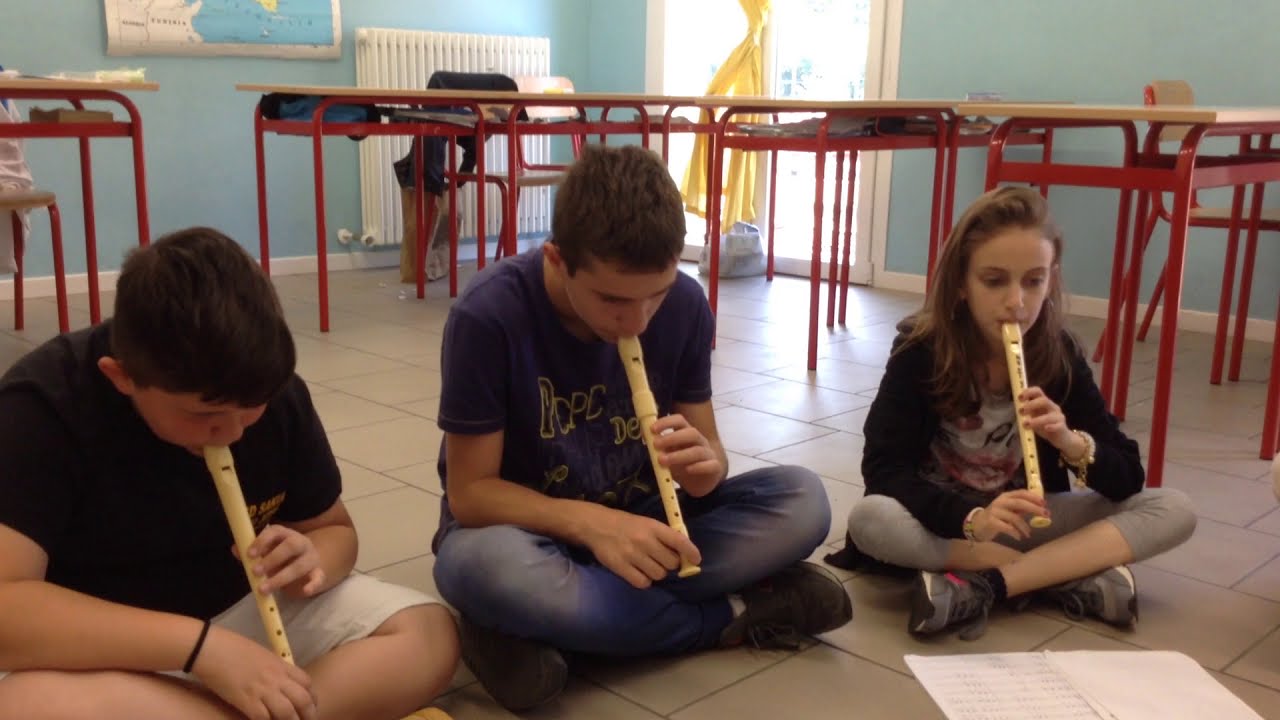In this photograph taken inside a classroom, three middle school-aged children—two boys and one girl—are seated cross-legged on a white tiled floor, each playing a cream-colored recorder. The boys, appearing taller and bigger, are positioned on the left, while the girl is on the right, attentively looking at an open sheet of music in front of her. The classroom background features a blue-painted wall with white trim, lined with desks that have red legs and tan tops. Additionally, there's a visible radiator, a partially seen map on the wall, and a sliding glass door through which bright white light is streaming in. The children are dressed in a variety of clothing: one in a white shirt with gray pants, another in a blue shirt with light blue jeans, and the third in a black shirt with white shorts. This image vividly captures a moment of musical practice amidst a typical classroom setting.